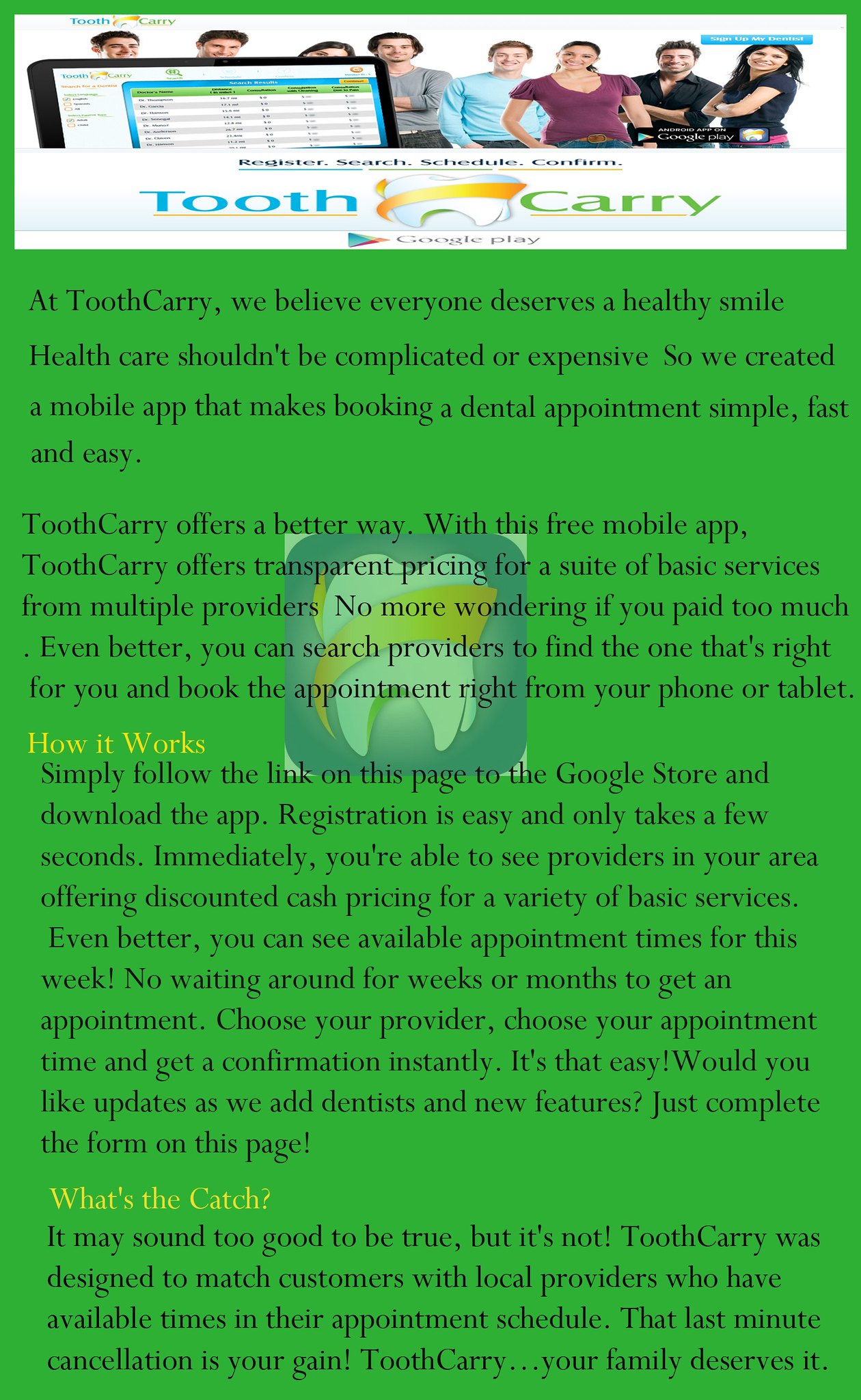The advertisement, likely for a dentistry service or app called "Tooth Carry," features a prominent green background adorned with several blocks of black text. At the top, there is a stretched and slightly distorted image that reads "Tooth Carry," with the word "Tooth" in blue font and "Carry" in green font. Above this text, a white rectangle displays seven or eight people standing together, with some faces obscured by what seems to be a computer screen.

In the center of the advertisement, there's an image of a tooth wrapped with something, partially transparent and overlaid with black text. This text champions the benefits of the Tooth Carry app, claiming, "At Tooth Carry, we believe everyone deserves a healthy smile." Detailed paragraphs explain how the app offers transparent pricing and a better way to manage dental health, encouraging users to download the app from the Google Store.

Additional sections feature headings in yellow, such as "How it works" and "What's the catch," with corresponding explanatory text beneath each heading, all in black Times New Roman font. While the design includes clipart elements and stretched images, the overall layout appears cluttered and poorly executed, focusing heavily on promoting the dentistry app.